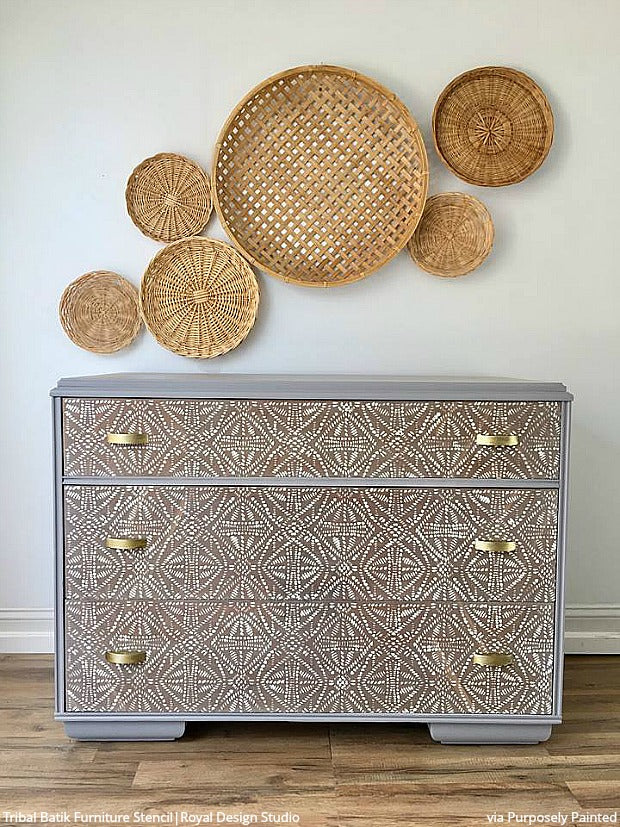This indoor scene captures a meticulously arranged living space featuring a light gray dresser adorned with six gold pull handles organized symmetrically on its three drawers. Above, a collection of intricately woven, circular trays made from hay or a similar straw material are artistically displayed on a white wall. These trays vary in size, with the largest positioned centrally and smaller ones situated in the upper right and bottom left corners. The wall is complemented by a white wooden molding at the bottom, meeting a floor of medium brown hardwood that has a slight grayish tint and consists of small planks. The dresser itself showcases a striking brown and white patterned stencil that evokes an African aesthetic. Adding a contemporary touch, textual elements are embedded in the image, with "Tribal Batik Furniture Stencil Royal Design Studio" in white on the bottom left and "VIA Purposely Painted" on the bottom right.